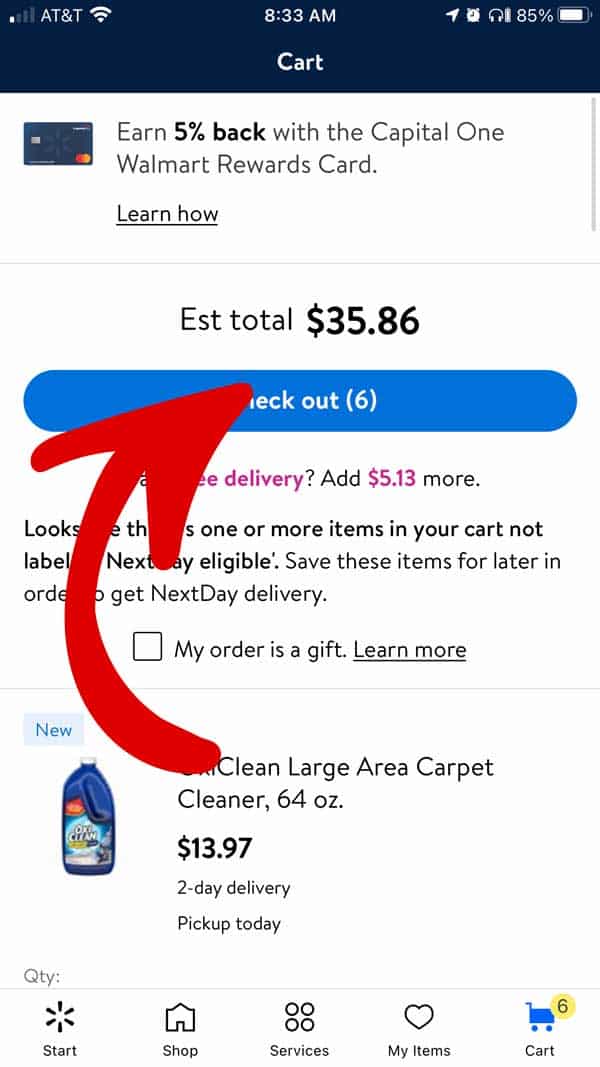**Caption:**
A mobile screenshot of a checkout page on a McCart shopping app, displaying several notable details. At the top left corner, the network provider is AT&T, and the screenshot was captured at 8:33 AM with the battery level at 85%. The header displays a blue background with the text "Cart" prominently featured. Below the header, a promotional message states, "Earn 5% back with the Capital One Walmart Rewards Card," accompanied by a clickable link labeled "Learn How." 

To the left, a visual representation of a rewards card is depicted, likely related to the promotion. Further down, the estimated total of the items in the cart is shown as $35.86. A blue checkout button indicates there are six items in the cart. Part of the screen is obscured by a large red arrow, directing attention to a notification that mentions some items in the cart are not eligible for next-day delivery and can be saved for later to avail of next-day delivery services. There is also an option to mark the order as a gift with a checkbox and a "Learn More" link for additional information.

Below the main text, an item is partially visible, showing a blue bottle cleaner with a white cap, labeled "Clean Large Area Carpet Cleaner, 64 ounces," priced at $13.97 with the availability of two-day delivery and an option for pick up today.